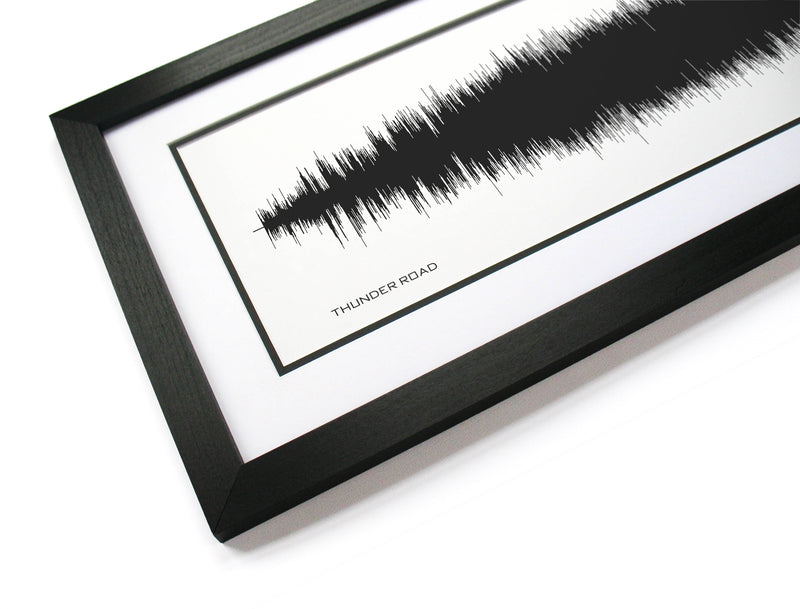This image showcases a modern framed piece of art, approximately 16 inches long, displayed on a white surface, possibly a table. The black picture frame encapsulates a white background with a central black waveform representing varying sound tones, reaching from low to high pitches. This waveform is likely an audio file visualization adorned with the text "Thunder Road" in small black letters beneath it. The white background is bordered by a thin black line, adding a sleek and modern touch to the artwork. The photo is taken at an unusual angle, hinting at a side perspective, creating visible shadows beneath the frame, suggesting it is resting on a flat surface. The overall minimalistic black and white color scheme enhances its contemporary aesthetic, making it a suitable piece for wall display.